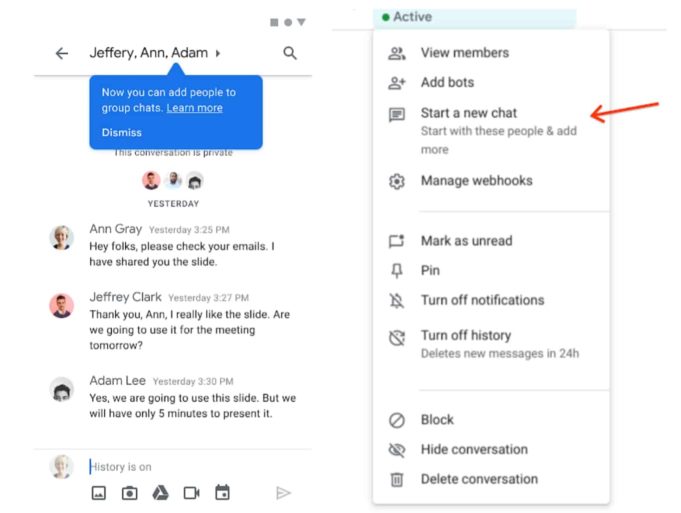**Detailed Caption:**

This image is a screenshot of a web or app-based chat interface. The layout is divided into two main sections: the left-hand side showing the conversation and the right-hand side displaying additional options.

On the left, there is a messaging thread involving three participants—Jeffrey, Anna, and Adam. A blue box points to a notice that reads, "Now you can add people to group chats," with options to "learn more" or "dismiss" this message. Below this, there is a privacy note stating, "This conversation is private," and it includes avatar icons for each participant. The conversation timestamp is marked "yesterday."

In the conversation, Anne Gray prompts the group by saying, “Hey folks, please check your emails. I have shared you the slide.” Jeffrey Clark responds with, “Thank you, Anne. I really like the slide. Are we going to use it for the meeting tomorrow?” Adam Lee adds, “Yes, we are going to use this slide, but we will have only five minutes to present it.” At the bottom, there's a prompt indicating that chat history is enabled, along with a text input area for further messaging.

On the right-hand panel, there is a dropdown menu headed by a blue bar labeled "active," featuring a green dot to signify the status. Below are various options for managing the chat, such as "View members," "Add bots," "Start new chat," "Manage webhooks," "Mark as unread," "Pin," "Turn off notifications," "Turn off history," "Block," "Hide conversation," and "Delete conversation." There’s a red arrow pointing specifically to the "Start new chat" option.